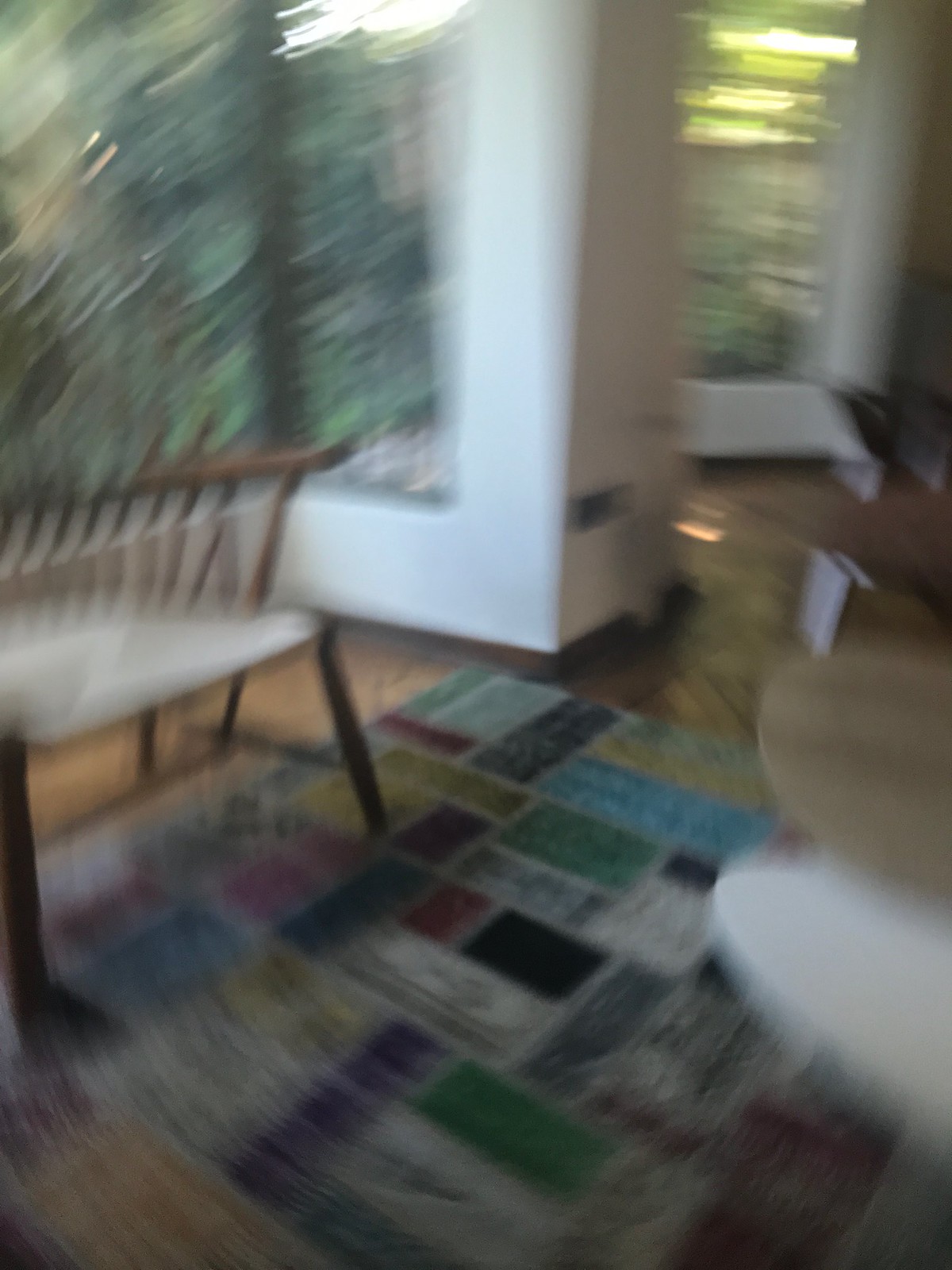The image depicts the interior of a room with a blurred focus. The floor is made of wood, and there is a large, colorful throw rug at the center. The rug features an array of colors including blue, green, black, gray, and burgundy arranged in patchwork patterns. On the left side of the room, there is a dark wooden bench with a white seat. The walls are painted white, and there is a large window on the left wall, allowing a view of greenery outside. A similar window appears in the background, also trimmed in beige. The ceiling appears to have lights installed. On the right side of the room, there is a wooden table, although the details are obscured by the blur. Scattered papers can be seen on the floor toward the upper right area of the image. The overall impression is one of a spacious and eclectic room, though the blurriness makes it difficult to discern finer details.